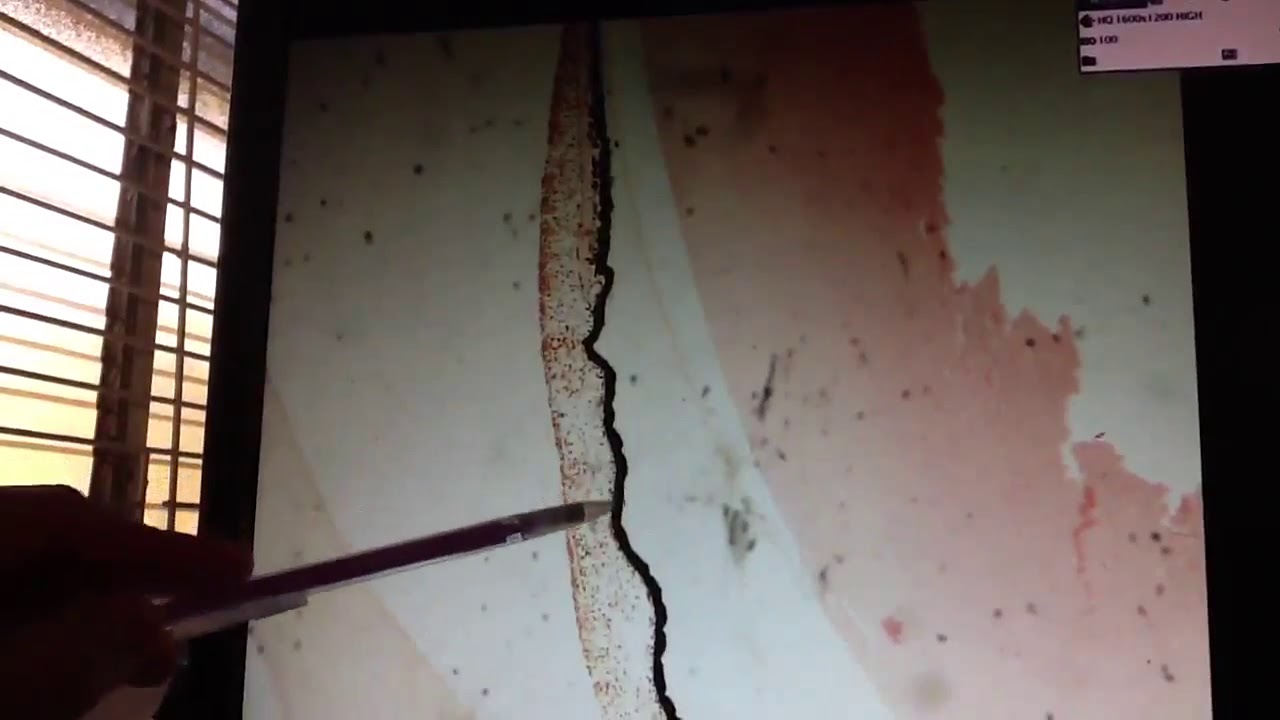The image is a horizontally-oriented photograph of an abstract painting with a predominantly white background. Splashes of pink paint are prominent in the center, with additional smaller pink streaks and splatters scattered to one side. A dark, irregular black line runs parallel to one of the smaller pink lines, adding contrast to the composition. A pen or similar object appears to be placed across or in front of the painting at an unusual tilt, suggesting it may be either taped to or resting against the canvas.

To the left of the image, there's a window with partially open blinds, divided by a beam that ends in a black element. The room is dimly lit, with most of the light coming from the window. Specifications such as speckles of red paint near the black line and a digital display with indistinct characters on the right add intricate details. Additionally, a faint hand gripping a stylus or pencil is visible, appearing to trace along a line on the painting. The indoor setting and the abstract nature of the artwork contribute to the overall complexity and intrigue of the scene.